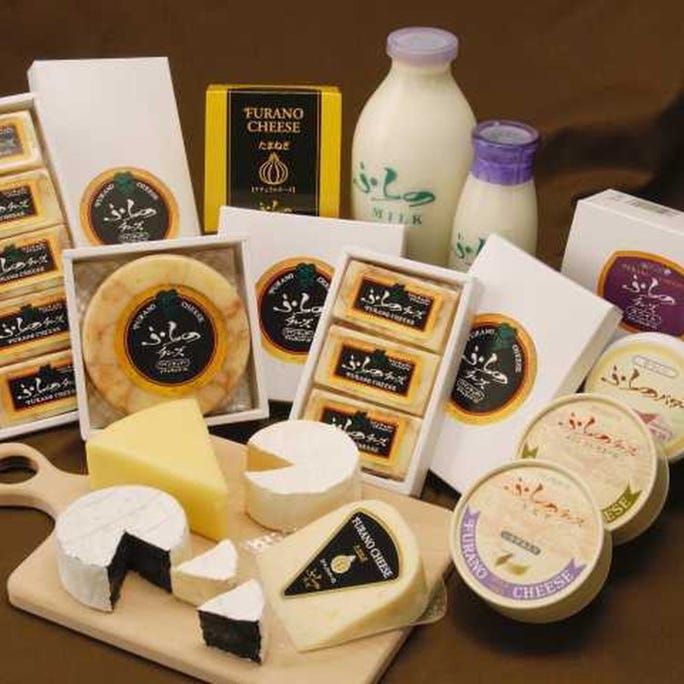This is a detailed frontal photograph showcasing a variety of Fiorano cheeses, arranged elegantly as if for an advertisement. Central to the display is a cheese board featuring small cheese wheels, some of which have wedges delicately cut out, alongside larger cheese wedges. In addition, there are circular and block-shaped cheeses in open cardboard boxes, with closed boxes nearby displaying enticing pictures of cheese. Bottles of Fiorano brand milk can be seen in the background. This professionally composed image, highlighting the luxurious quality of the cheeses, suggests that they are potentially expensive and gift-worthy.